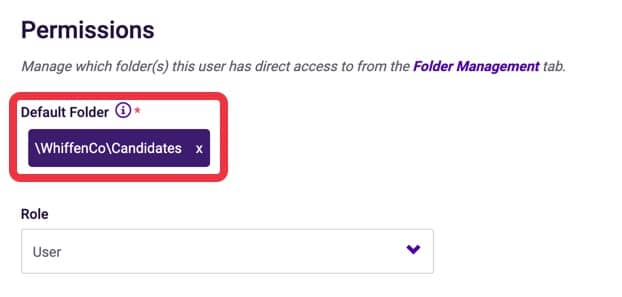This image is a cropped screenshot focusing on the "Permissions" section of a user interface. Spanning the top left corner, the word "Permissions" is displayed in a bold, purple font. 

Below this heading is an italicized caption reading, "Manage which folders this user has direct access to." This is followed by another bolded purple heading stating "Folder Management." Beneath this, there is a section titled "Default Folder" marked by a red asterisk, accompanied by an information icon. 

To the right of this section, prominently featured within a thick red border for emphasis, is a purple rectangular button filled in with white text that reads "dash within code dash candidates." A white 'X' is situated next to this button. 

Further down, another bolded heading reads "Role." Adjacent to this is a longer rectangular drop-down menu with the word "User" filled in, and a purple drop-down button to its right. The thick red border surrounding the "Default Folder" section suggests that this area is particularly important and requires user attention, possibly as part of a tutorial or guided workflow.